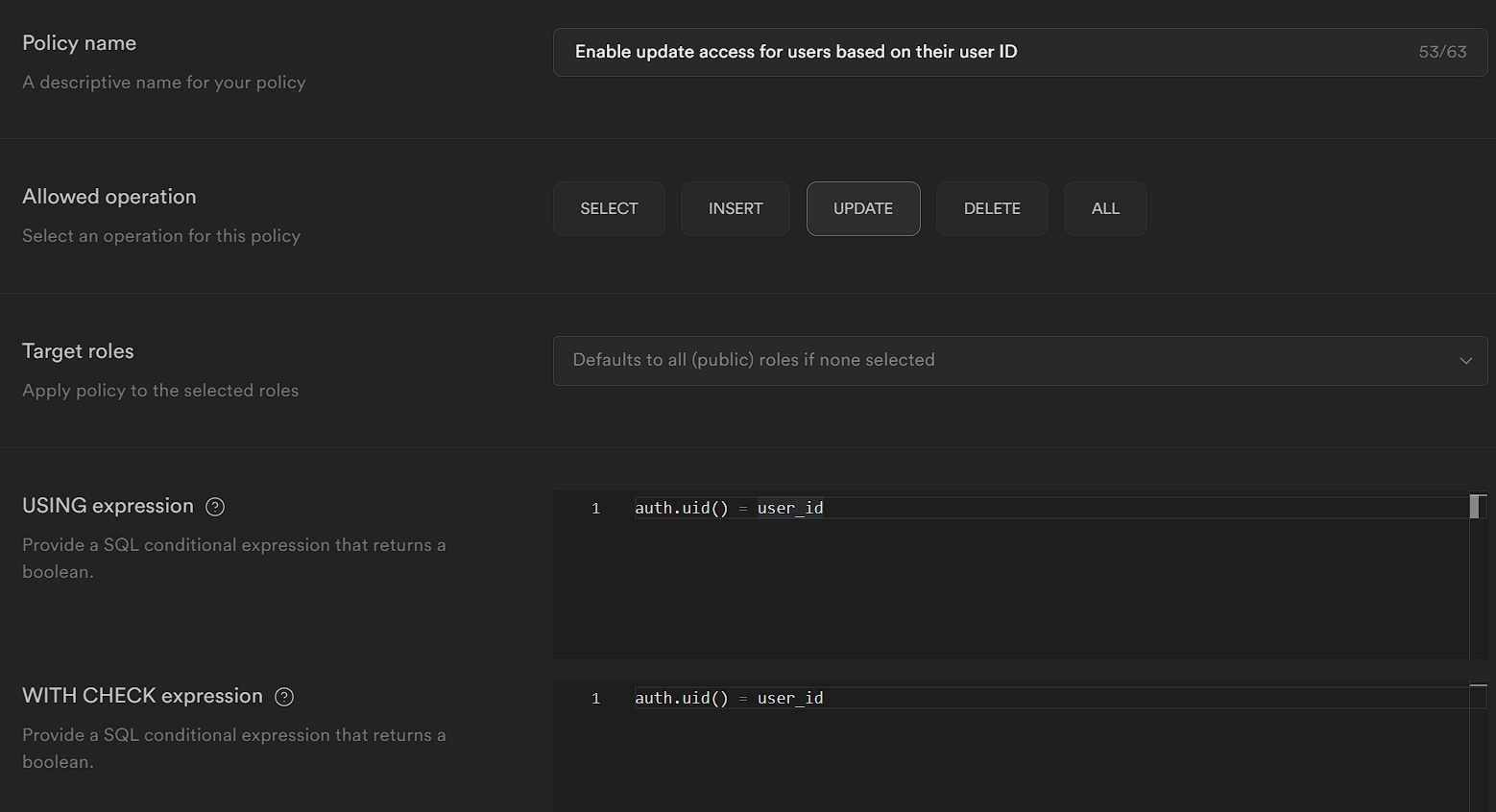This cropped screenshot displays an access panel for an administrative permissions software, set against a black background. In the top left corner, the text "Policy Name" is displayed in small, white, bold font. Directly below this, there is the prompt "a descriptive name for your policy." Further down, the text "Allowed Operation" appears, followed by "select an operation for this policy". Then "Target Roles" is listed, under which the instruction "apply policy to the selected roles" is given. Continuing downward, "Using Expression" is seen, succeeded by "provide SQL conditional expression that returns a Boolean". At the bottom left, "With Check Expression" is written, adjacent to "provide SQL conditional expression that returns a Boolean".

On the right side of the screenshot, at the top in bright white letters, the directive "Enable update access for users based on their user ID" is prominently displayed. In the top right corner, "53 out of 63" indicates the current status of role application. Below this, five selectable boxes are labeled "Select", "Insert", "Update", "Delete", and "All". Further down, a lengthy drop-down box is visible, currently set to default "to all public roles if none selected". Below this dropdown, there are two large text boxes designated for code input. The first text box contains "auth.uid", and then in parentheses, "- user_id".

This clean and detailed annotation retains all essential elements of the interface, enhancing clarity and understanding for users navigating the software.